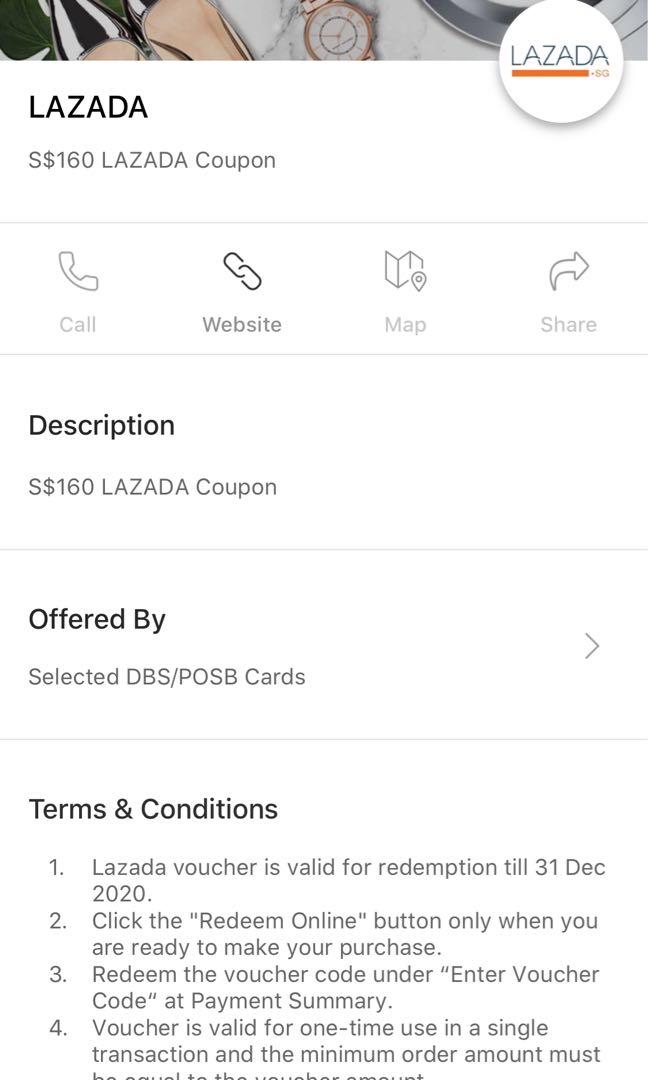Lazada $160 Coupon Promotional Offer (Lazada SG).

This promotional offer features a $160 coupon for use on Lazada, valid exclusively with selected DBS/POSB cards. The offer details and terms include:
1. The Lazada voucher is valid for redemption until December 31, 2020.
2. Click the 'Redeem Online' button only when you are ready to make your purchase.
3. Enter the voucher code at the payment summary under the 'Enter Voucher Code' section.
4. The voucher is valid for a one-time use in a single transaction, with a minimum order requirement (details cut off).

The visual above the description includes an image strip, prominently displaying a watch with a copper-colored metal frame. The Lazada logo is shown in a combination of blue and gold/orange colors against a background featuring black, gray, and white shades.

Visual indicators accompanying the offer include icons representing:
- Call (depicted by a phone symbol),
- Website (depicted by two linked icons),
- Map (depicted by a folded map),
- Share (depicted by an arrow pointing to the right).